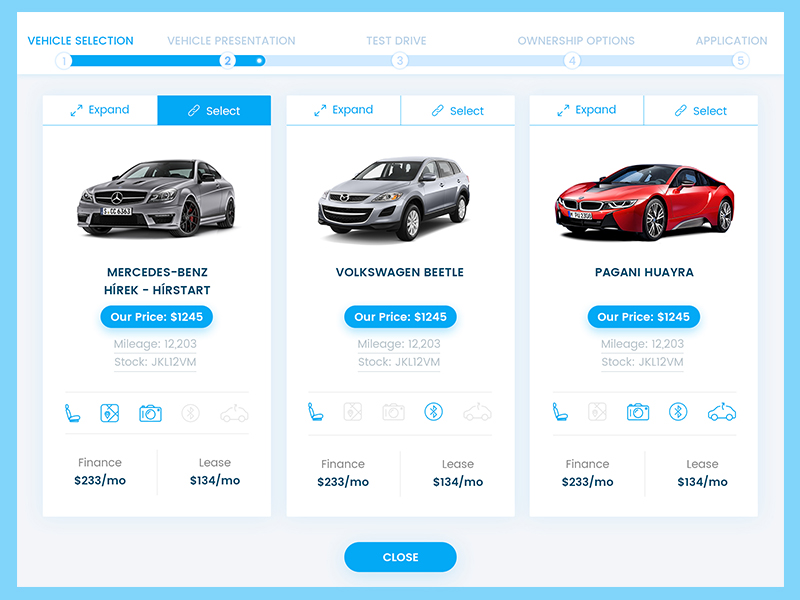The image depicts a structured layout with a blue-bordered white box. At the top, there is a sequence of headings each followed by a number, specifically: "Vehicle Selection (1)", "Vehicle Presentation (2)", "Test Drive (3)", "Ownership Options (4)", and "Application (5)". Below these, there are three distinct sections.

The leftmost section labeled "Expand and Select" showcases a gray or silver Mercedes-Benz. Detailed specifications of this vehicle include:
- Price: $1,245 
- Mileage: 12,203 miles
- Stock Number: JKL12VM
- Financing Option: $233 per month
- Leasing Option: $134 per month

Next to this, there is information on a Volkswagen Beetle, listing:
- Price: $1,245 per month
- Mileage: 12,203 miles
- Stock Number: JKL12VM

The overall layout provides a comprehensive overview of vehicle selection and financial options available for prospective buyers.